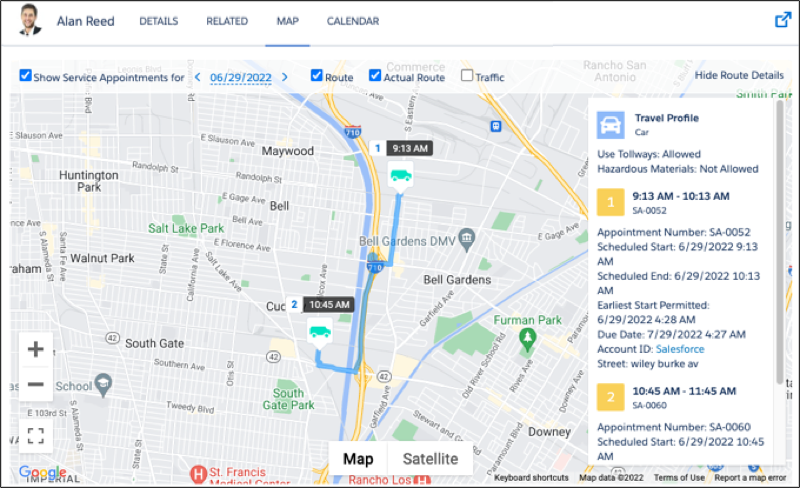In this screenshot image, we see a detailed map outlined in thin black lines, highlighting specific areas within a rectangular frame. In the upper-left section of the screenshot, there is a smaller inset featuring a young man's face with the name "Alan Reed" displayed to the right. 

The map below this section is underlined in blue, signifying an active status or important detail. Clearly visible above the map, there is a header that reads "Show service appointments for 6-29-2022," marked with a checkmark in a blue box, indicating completion or confirmation. Additionally, to the right of this header, there are checkmarks next to labels that indicate the planned route and the actual route have been confirmed.

On the map itself, specific times for scheduled appointments are noted: "9:13 a.m." and "10:45 a.m." The map also identifies prominent locations and areas including Huntington Park, Walnut Park, Maywood, Bell Gardens, Downey, and St. Francis Medical Center. The combination of these details illustrates a schedule and route for service appointments on that particular date.